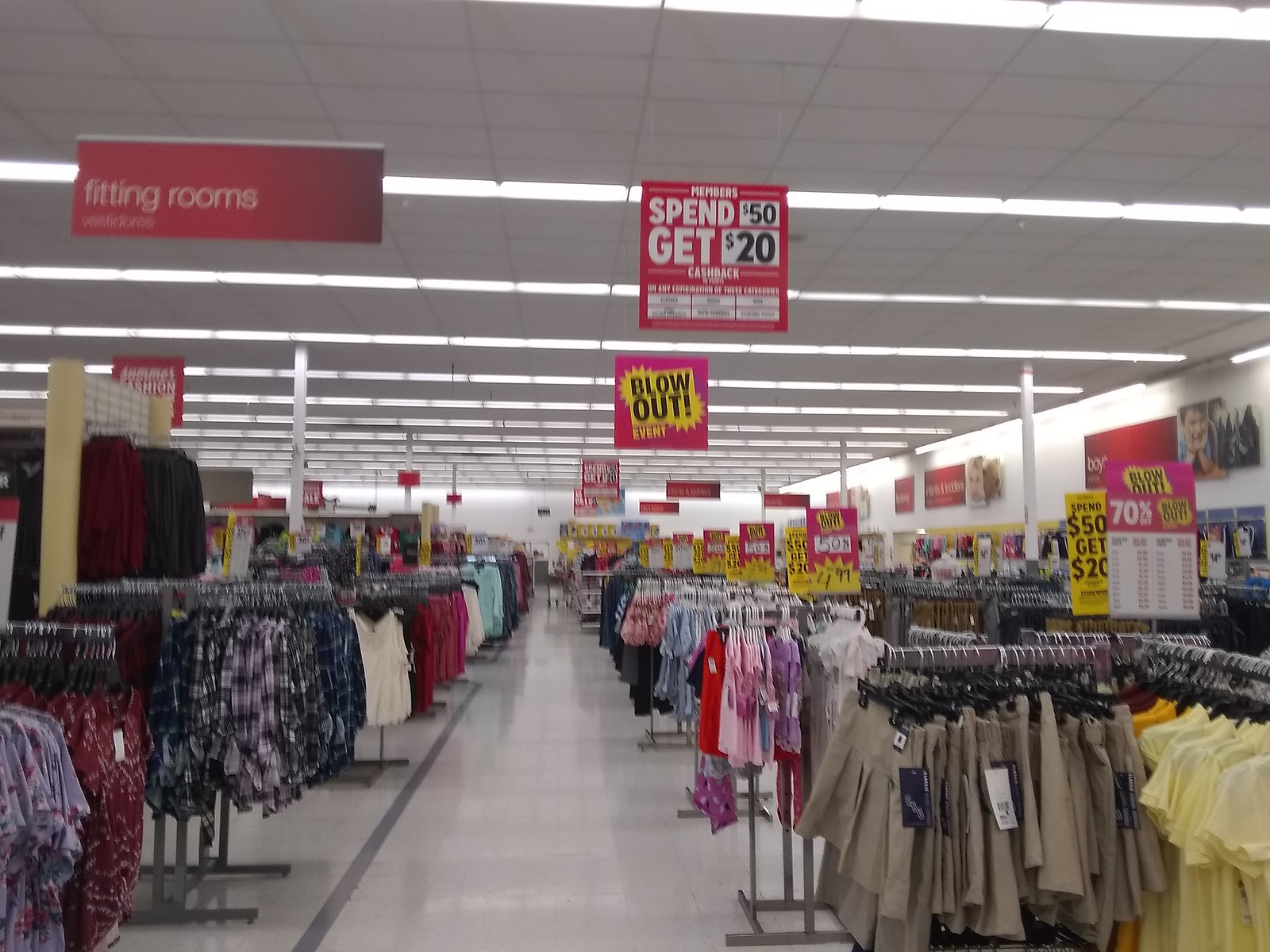The image depicts the interior of a low-cost clothing store, featuring a section dedicated to uniforms prominently at the front. The uniforms include khaki pants and skirts, with light yellow, dark yellow, and red shirts, suggesting it may be the girls' section. Beyond the uniforms, the store is organized into rows of diverse clothing options ranging from pajamas to flannel shirts in various colors, indicating a wide range of affordable apparel.

Signage throughout the store advertises significant discounts, including a blowout event with items marked at 50% and 70% off, and specific racks priced at $4.99. A promotional banner overhead promises members $20 cash back for spending $50, although other details on the banners are too blurry to discern. To the left, fitting rooms are available for trying on clothes. The aisle running down the center of the image is clear of shoppers, suggesting a quiet moment, with possibly a store worker seen towards the back.